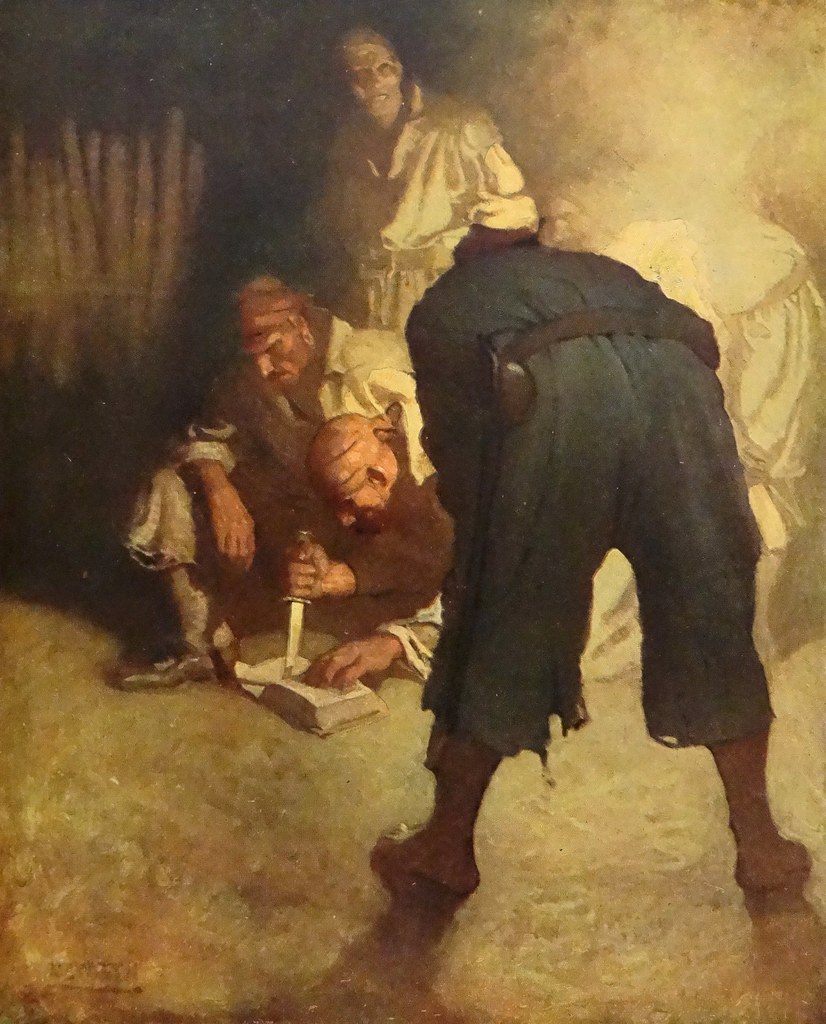The painting depicts a dimly lit indoor scene resonant with the aesthetic of Renaissance artworks, featuring dark hues of yellow, gray, and green. A group of four men, possibly pirates dressed in period-appropriate attire—baggy pants, belts, and bandanas—are engrossed in an enigmatic act involving a book. The central figures, hunched over the book illuminated by a mysterious light source that heavily contrasts with the surrounding darkness, seem to be plotting something. One man, barefoot and in ragged clothing, is prominently seen from the back, his hand steadying a knife poised to cut through the book's pages. Another man nearby aids him, his gaze fixated on the book. In the background, a third man's face is harshly highlighted by the light, while a fourth man stands partially obscured, possibly peering at the book as well. A faint signature, barely discernible, is located in the bottom left corner of the painting, hinting at the artist's hidden identity.